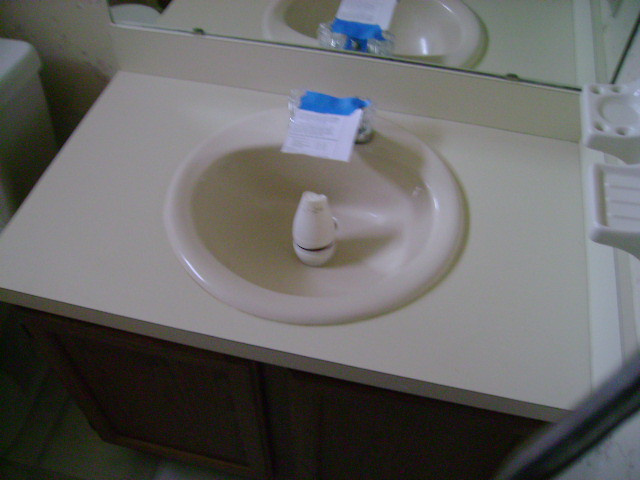A close-up, landscape-oriented photograph captures a bathroom sink and its surrounding details, albeit in a somewhat grainy, low-resolution manner. The sink, situated in the center of the image, features a white countertop and a porcelain bowl. Inside the sink, there is a cylindrical, twist-open air freshener without a visible brand label. The freshener is slightly open, revealing a dark-colored content inside. Near the sink handles and knobs, a piece of white paper with blue tape suggests the sink may need testing or repairs. 

In the background, the upper right-hand corner shows soap dishes and a mirror. Below the sink, wooden textured storage doors are visible. To the left, the partially out-of-focus image includes the tank and lid of a toilet, positioned against a yellow, possibly stained or dirty wall. The floor appears to be greenish, though the focus is too poor to confirm this detail accurately.